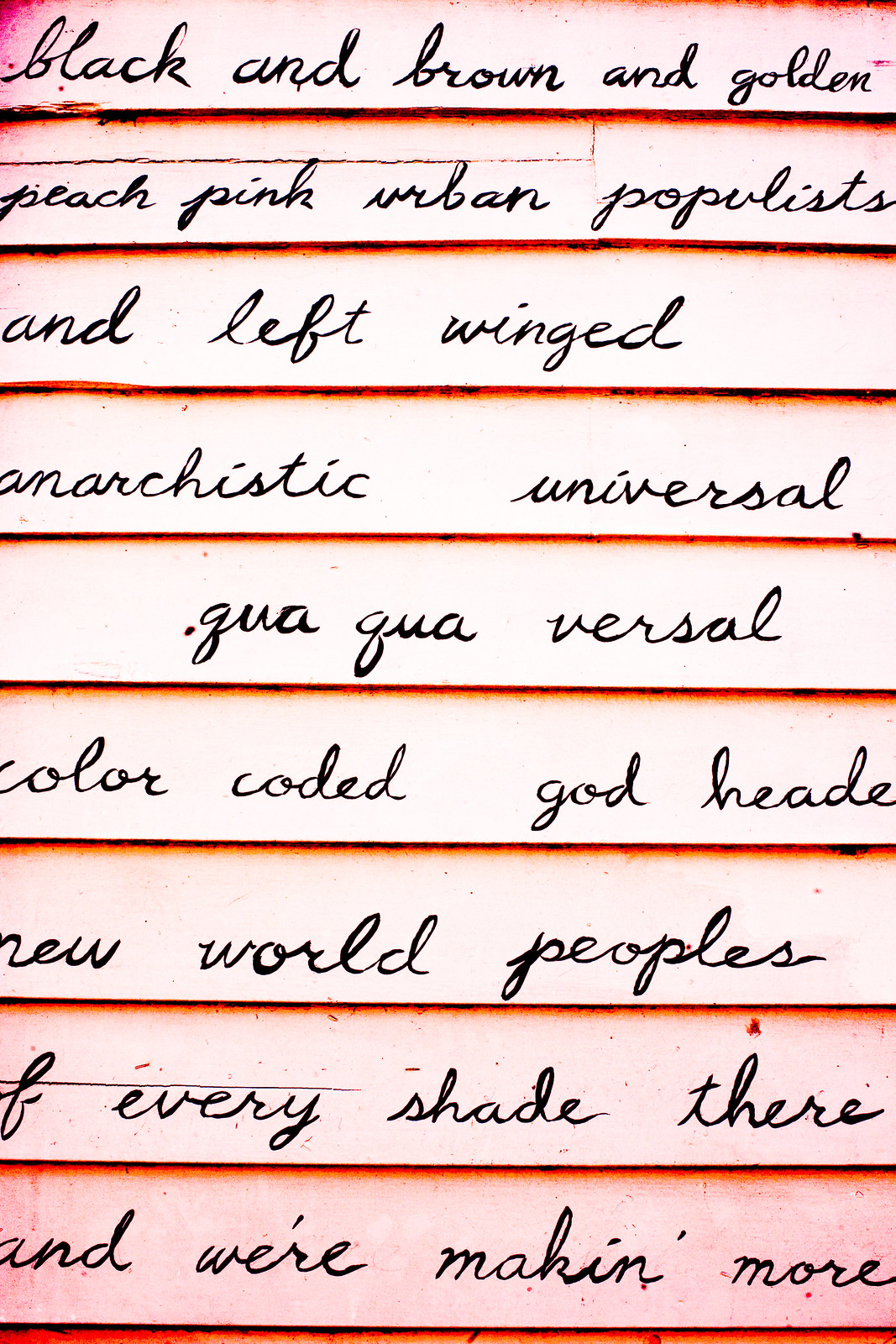The photograph shows a close-up of handwritten text in black ink on what appears to be the side of a house, likely white but tinted pinkish due to lighting conditions. The text, which dominates the image, reads: "Black and Brown and Golden, Peach, Pink, Urban Populists and Left-Winged, Anarchistic, Universal, Qua-Qua-Versal, Color-Coded, God-Headed, New World Peoples. We have every shade there, and we are making more." The handwriting seems to have a red horizontal underline beneath each sentence, although some parts of the text might extend beyond the photograph's frame. There are no other discernible objects in the image, making the text the focal point. The bright natural light enhances the visibility and clarity of the text, giving the overall impression that the message is intended to be motivational or inspirational, something one might see circulating on social media.